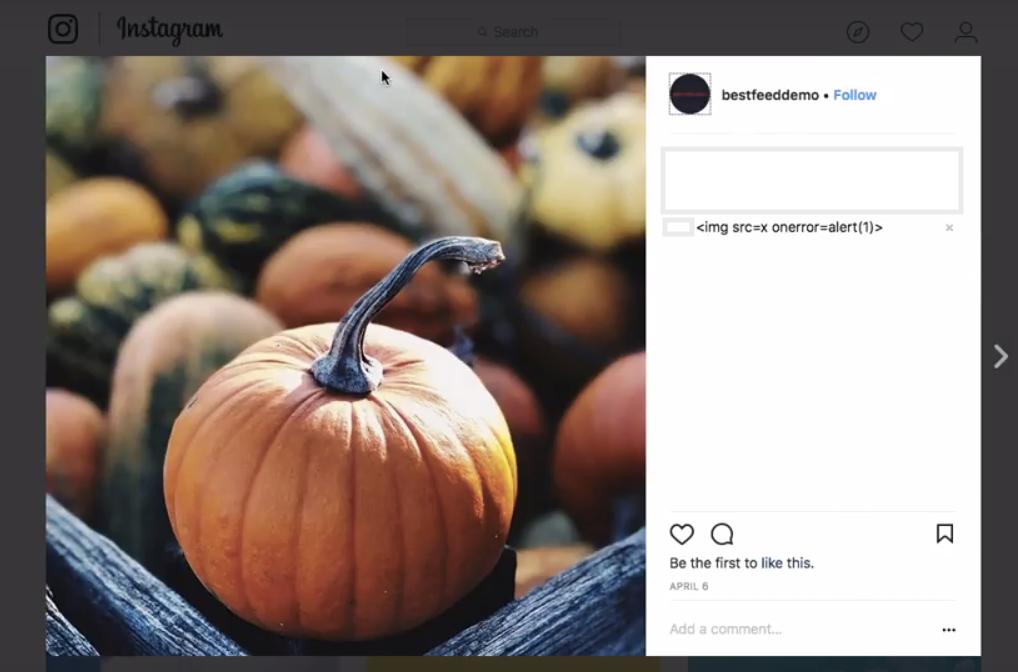The image features a black background with a large, visually striking blue wooden crate prominently displayed on the left side. Inside the crate, a variety of pumpkins are arranged, creating an autumnal scene. The centerpiece is a vibrant orange pumpkin with a distinctive greenish-black stem. Surrounding it, there are pumpkins of various shades, including green, brown, red, yellow, and another long white gourd with a small black arrow pointing upward.

On the right side of the image, there is a sizeable white box containing several elements. At the top, a smaller box features a black circle with the text "Best Feed Demo," followed by a blue "Follow" link. Beneath this is a section with blue outlined boxes and some code-like text, which reads: "more than, IMG, SRC, equal X, on arrow, equal alert, (1), right arrow, and X."

Further down, there are icons for a heart and a conversation box. A partial ribbon overlays the right side, reading "Be the First to Like This." Below it are the details "April 6th" and an "Add a Comment" box accompanied by three little dots, and a right-pointing arrow within a black outline on the rightmost side.